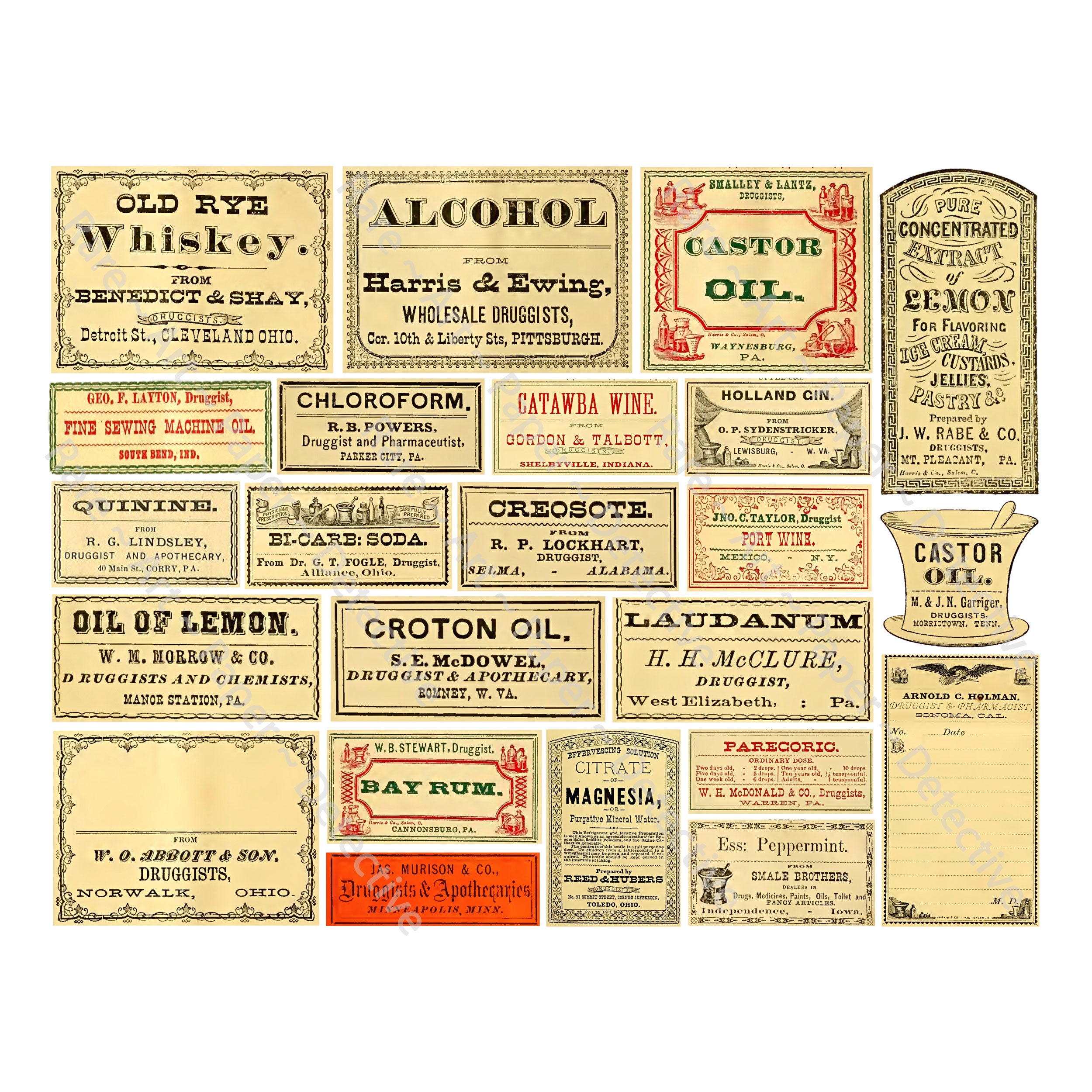The image features a meticulously arranged collection of vintage medicinal product labels from the late 1800s to early 1900s, showcasing the nostalgic charm of old-timey fonts, hues, and designs. Predominantly in a vintage cream color with black print and occasional red accents, these labels represent an array of pharmaceuticals and remedies such as Old Rye Whiskey, Castor Oil, Chloroform, Oil of Lemon, Croton Oil, Bay Rum, and both Citrate and Magnesium. Authenticity is suggested by the inclusion of historical pharmaceutical company names like Harrison Ewing, Wholesale Druggist, and RB Powers Druggists and Pharmaceuticals. Other notable labels include Fine Sewing Machine Oil, Catawba Wine, Holland Gin, Laudanum by H.H. McClure, and several from W.O. Abbott & Son and various druggists from locations like Norwalk, Ohio, and Romney, West Virginia. This collection serves as a fascinating window into the past, reflecting the medical practices and marketing styles of turn-of-the-century America.